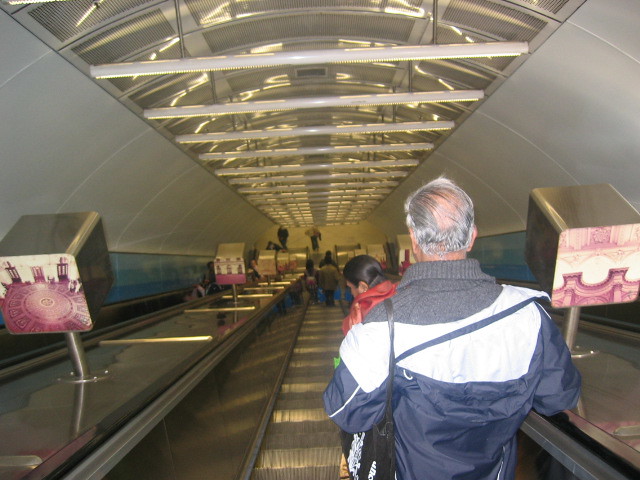The photograph captures a man at the top of a descending escalator, set within a tunnel-like structure with gently curving walls that transition from white to blue. He is positioned at the center and gazes downward, with two additional individuals directly below him—a man with silver, balding hair who wears a white and blue jacket paired with a gray sweater, and a woman with brown hair in a red jacket. Further down the escalator, more people are seen standing, waiting to descend, while on the adjacent left escalator, individuals can be observed ascending. The surrounding environment of the escalator tunnel includes a tan-colored grated ceiling accented with fluorescent tube lighting and box-shaped displays featuring images of buildings or murals at intervals along the way. The central escalator, composed of silver metal stairs, is flanked by two similar units, each marked by reflective metal dividers. The configuration leads to a flat, white flooring at the bottom, indicating the end point of the descent.